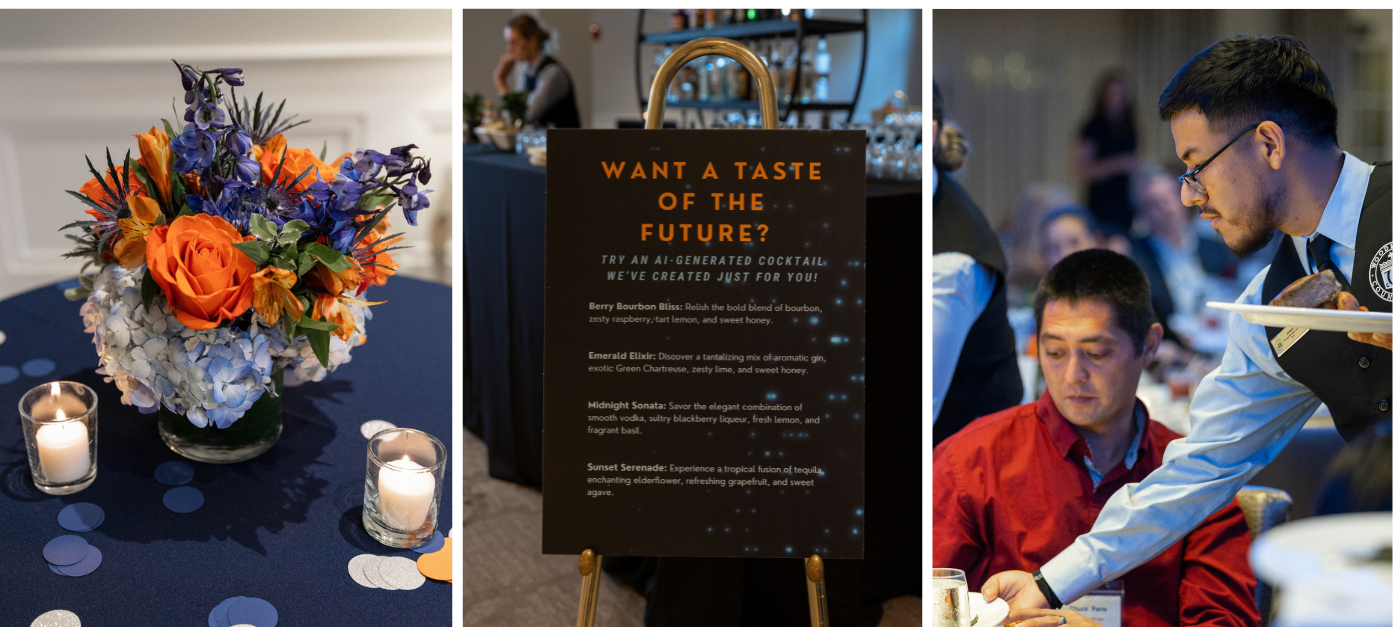This photo collage comprises three distinct images arranged side by side. The left image captures a circular table adorned with a vivid blue tablecloth. Centered on the table is a floral arrangement featuring orange, blue, and purple flowers. Flanking the arrangement are two lit candles in glass holders, and scattered across the table are blue and white circular chips. The backdrop is a plain white wall. The middle section of the collage features a promotional sign with the heading "Want a Taste of the Future?" positioned in front of what looks like a bar setup. The sign lists AI-generated cocktails such as Berry Bourbon Bliss, Emerald Elixir, Midnight Sonata, and Sunset Serenade, and there are blue tablecloths and racks of drinks visible behind it. To the far right, a bustling restaurant scene unfolds with a waiter in a blue collared shirt, tie, and black vest. The waiter, who has black hair and glasses, is serving a man in a red long-sleeve shirt. The man sits among other patrons, indicating a lively atmosphere.